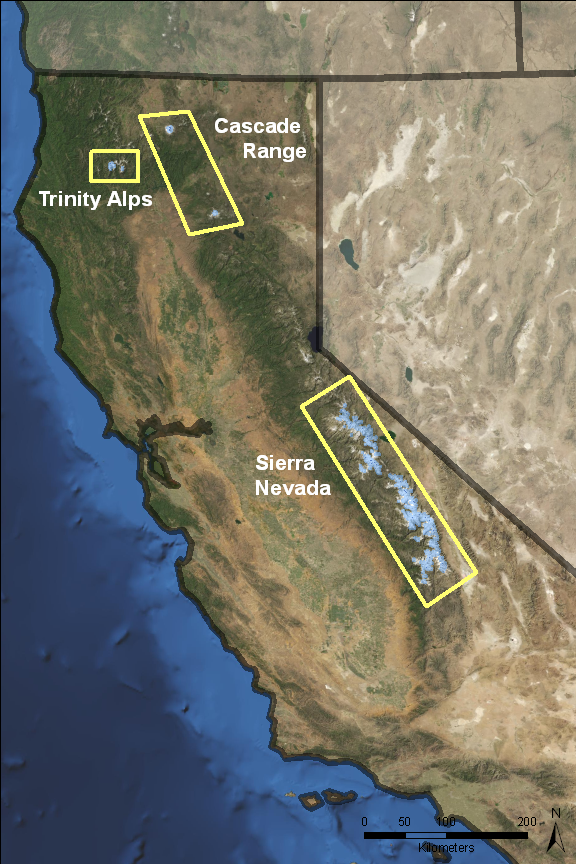This vertically aligned rectangular image is a detailed topographic map, predominantly showcasing the state of California with a part of the left side of Nevada visible in the upper right corner. The map highlights several key mountain ranges in California, including the Sierra Nevada, which is centrally located and marked by a yellow outline with its name printed to the left. 

Above the Sierra Nevada, another rectangular section is outlined, marking the Cascade Range in white text, situated in the upper central part of California. Further left of the Cascade Range, a smaller yellow-outlined rectangle highlights the Trinity Alps, also labeled in white. The map uses various shades of brown (medium, light, and dark) to represent different elevations, with the Sierra Nevada appearing in gray. California's coastline features shades of blue and darker blue representing water bodies, especially prominent in the lower left corner.

At the bottom of the image, a scale bar indicates distances in kilometers, starting at zero and extending beyond 50 to a total of 200 kilometers. The overall depiction emphasizes the natural topography, showing mountains, deserts, and water bodies in vivid detail while focusing primarily on California's geographic features.